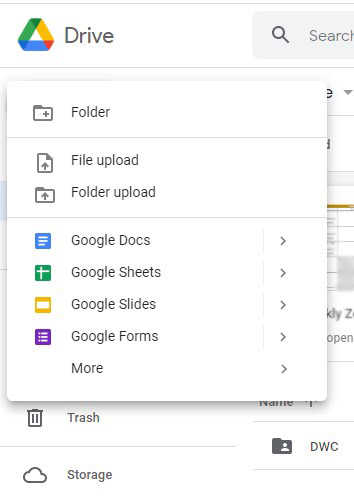In the image depicting a webpage, the background is entirely white. At the top, the familiar triangular logo of Google Drive is visible with a search bar featuring a magnifying glass icon. A pop-out menu is displayed prominently at the top. It lists various options with accompanying icons: 
- "Folder" represented by a file folder icon
- "File Upload" shown with a folded paper icon
- "Folder Upload" again with the file folder icon
- "Google Docs" illustrated by a blue square with white lines
- "Google Sheets," depicted as a green square with intersecting vertical and horizontal white lines
- "Google Slides," characterized by a white area with yellow stripes at the top and bottom
- "Google Forms," marked by a purple area with white lines and bullet points.

Each option has a right-facing arrow indicating further actions can be taken. 

Below this pop-out menu, part of the webpage is visible. Notably, there is a trash can icon and a cloud icon symbolizing storage. Additionally, a file folder named "DWC" is displayed.